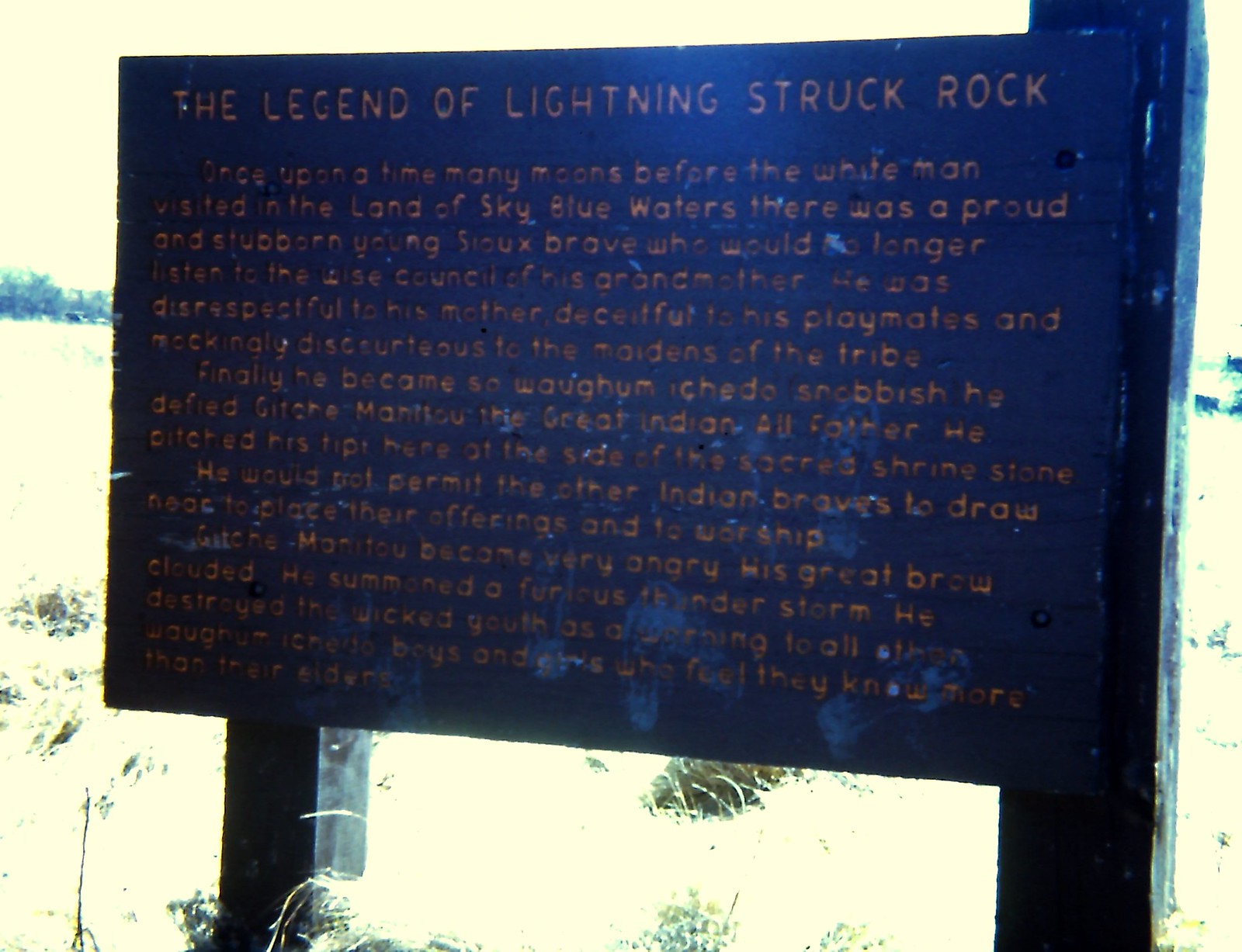This image displays an old, weathered plaque titled "The Legend of Lightning Struck Rock." The plaque is black with brown lettering, though some of the text is worn and hard to read. It is located outdoors in a sunny area. The tale begins with, "Once upon a time, many moons before the white man visited the land of the sky-blue waters, there was a proud and stubborn young Sioux brave who would no longer listen to the wise counsel of his grandmother." The narrative continues about the brave's disrespect towards his mother and deceitfulness towards his playmates, as well as his discourteous behavior towards the maidens of his tribe. The plaque recounts how he became so arrogant that he defied the great spirit and would not allow other Indian braves to make their offerings. The text is partially obscured due to age, making some sections difficult to decipher. The plaque suggests that the story is related to a rock nearby.